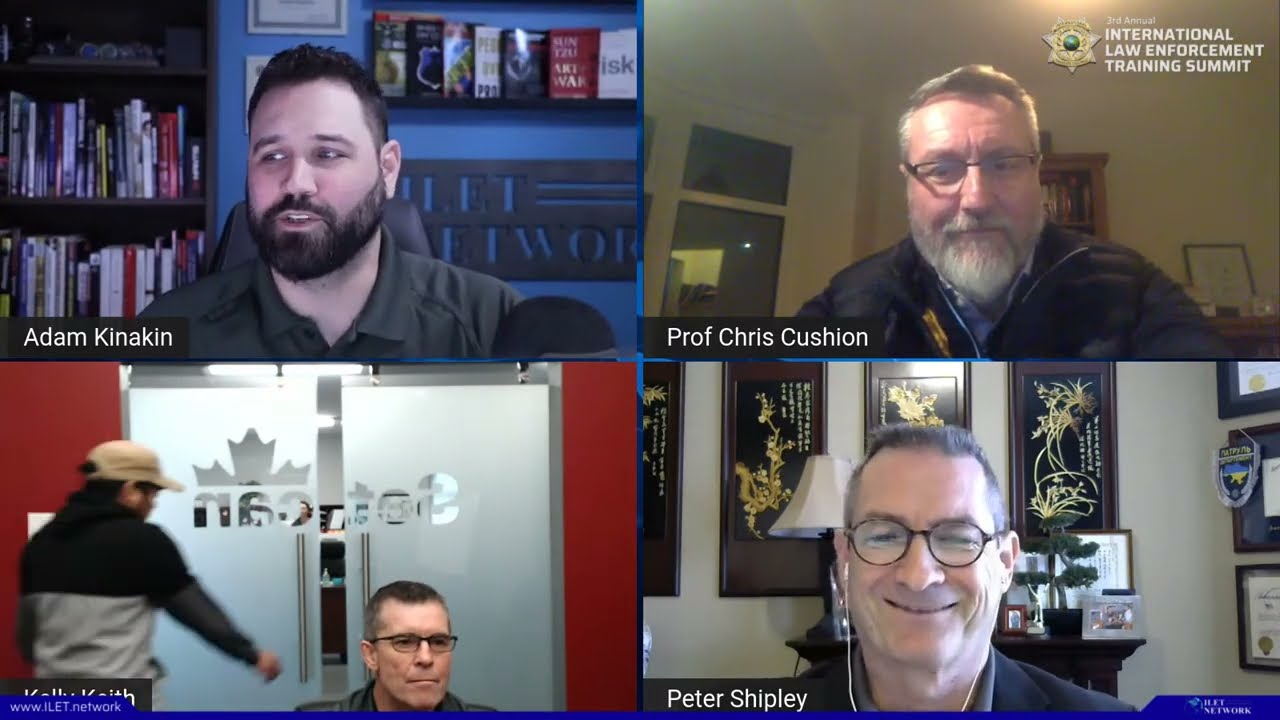This image is a screenshot of a Zoom or online conference call, featuring four participants each in a separate quadrant.

In the upper left quadrant, Adam Kinnikin is visible. He appears to be in his 40s with a full black beard and mustache, short black hair, and is wearing an olive green collared shirt. Behind him, there is a bookshelf on the left and another stack of books on the right. His name is displayed in white text on a black bar at the bottom left of this section.

The upper right quadrant shows Prof Chris Cushion seated at a desk. He is an older Caucasian man, probably in his 50s. He has gray hair, a full gray beard and mustache, and is wearing wire-rim glasses and a dark jacket. The background has a white wall with a bookshelf on the left and some framed items including a window on the right side. The top right corner features a logo with white text reading "International Law Enforcement Training Summit." His name is also displayed in a black bar with white text at the bottom left of this section.

In the lower left quadrant, a middle-aged Caucasian man with dark hair and dark-rimmed glasses is visible from the chin up. He is seated in a room with red walls and white double doors behind him, featuring a maple leaf logo and some backwards text. Another man in a gray and black striped hoodie and a baseball cap is visible in the background, appearing to leave the room. The name in the black bar at the lower left corner is partially obscured by a blue tab, making it unreadable.

The lower right quadrant features Peter Shipley, an older man who is also likely in his 50s or early 60s. He has short dark gray hair, round brown glasses, and an earbud in his right ear. He is smiling and is clean-shaven. The background shows a beige wall with multiple framed plaques and there is a stand with small plants and objects behind him. His name is displayed in white text on a black bar at the bottom left of this section.